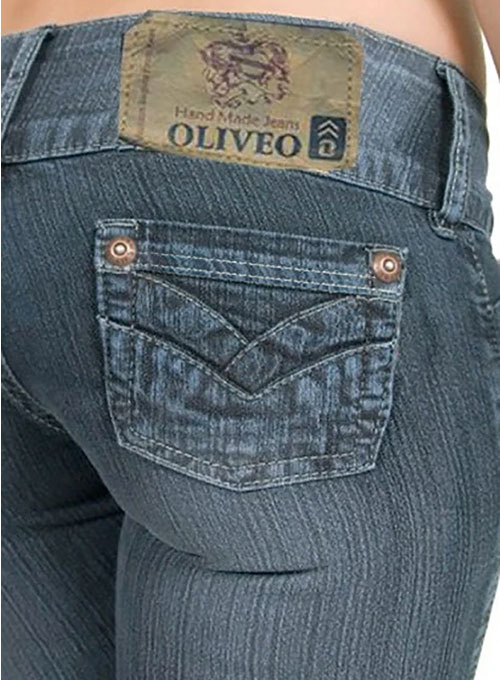The image appears to be an advertisement for Olivio handmade jeans, showcasing a three-quarters rear view of a model wearing very tight blue jeans. The focus is on a tan tag stitched above the right rear pocket of the jeans. The tag prominently features "OLIVIO" in navy blue capital letters beneath the words "handmade jeans" in maroon font, with some sort of insignia above the text. The jeans' design includes rust-colored buttons on the pockets, which have a narrow, decorative V-shape rather than being functional. The model is shirtless, though the photo only reveals up to the edge of the waist, clearly highlighting the snug fit and the curve of the jeans. The belt loops appear wide, adding to the detailed craftsmanship of the garment.